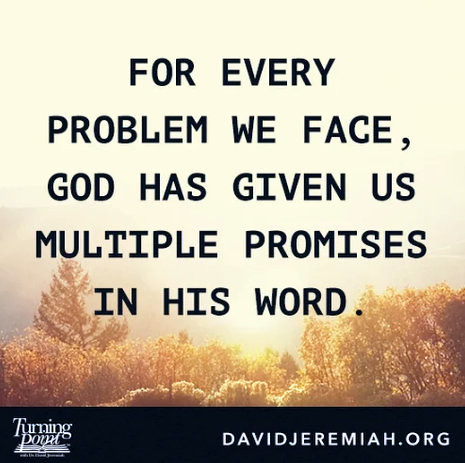The image features a poster prominently displaying the motivational message: "For every problem we face, God has given us multiple promises in His word," in bold black letters centered over a scenic background. The background depicts a peaceful wooded area bathed in a golden yellowish-brown hue, likely illuminated by sunlight, suggesting an outdoor setting in the middle of the day. Above the trees, the sky appears almost white due to the bright sunlight. At the bottom of the poster, a black strip runs across the image. On the lower left side of this strip is the logo "Turning Point," and on the lower right side, in white lettering, it reads "DavidJeremiah.org." The overall tone of the image is serene and inspirational, combining elements of nature with a religious and motivational message.